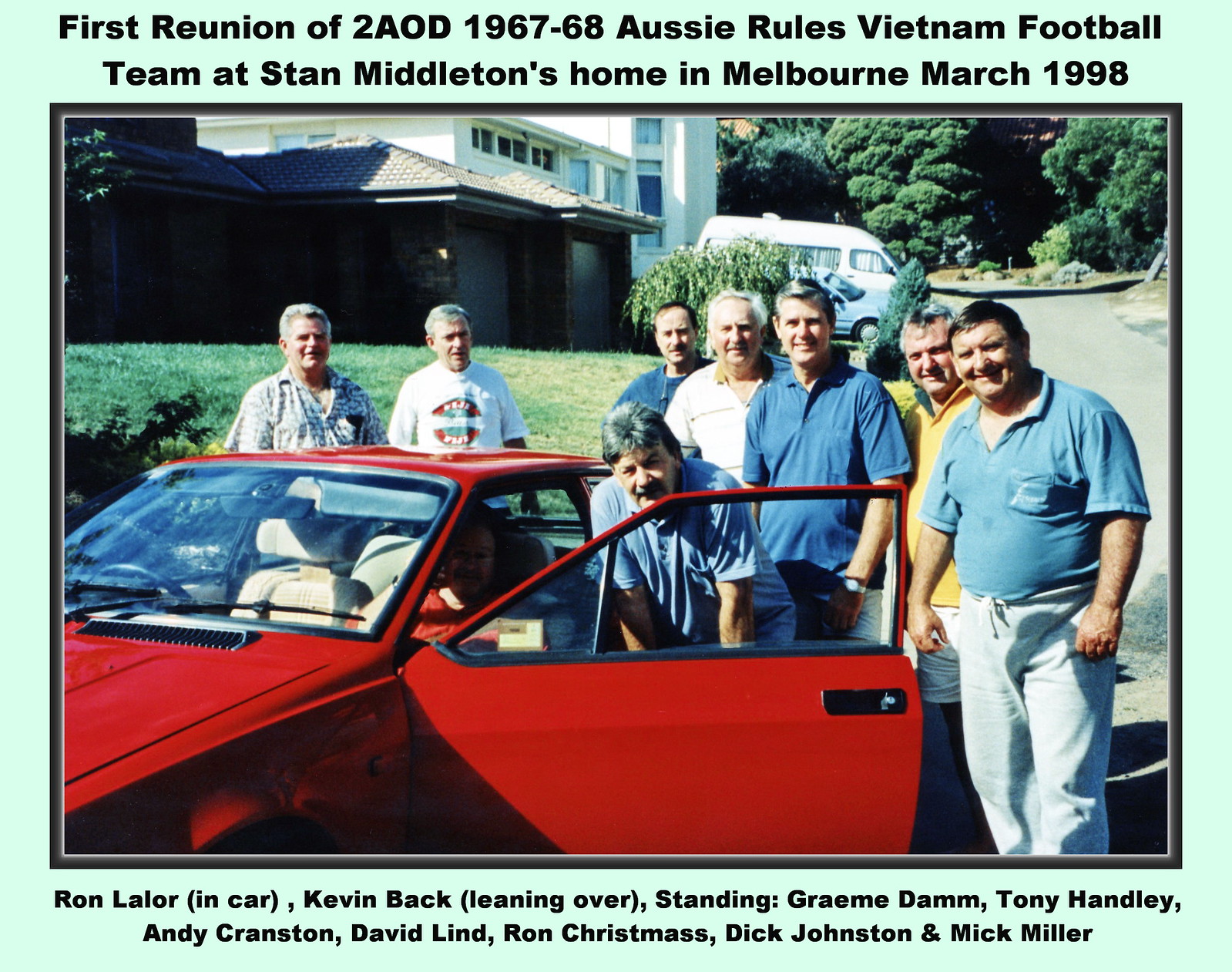This color photograph, encased in a light green border, captures a nostalgic moment from the "First Reunion of the 2AOD 1967-68 Aussie Rules Vietnam Football Team at Stan Middleton's home in Melbourne, March 1998." The center of the photo shows a red sedan with its door ajar, angled towards the left-hand corner. In and around the car are nine older white men, likely in their 60s, posing for the camera. Ron Layler is situated inside the car, while Kevin Back is leaning over, and the remaining men—Graham Dam, Tony Handley, Andy Cranston, David Lind, Ron Christmas, Dick Johnston, and Mick Miller—stand in a line, some slightly bent over. They are all dressed in different colored t-shirts and trousers, smiling, with white hair and a bit of a paunch. The backdrop includes a large house featuring a brown garage, a white facade, a minivan, and surrounding greenery. The idyllic setting adds to the charm of this reunion captured in March 1998.